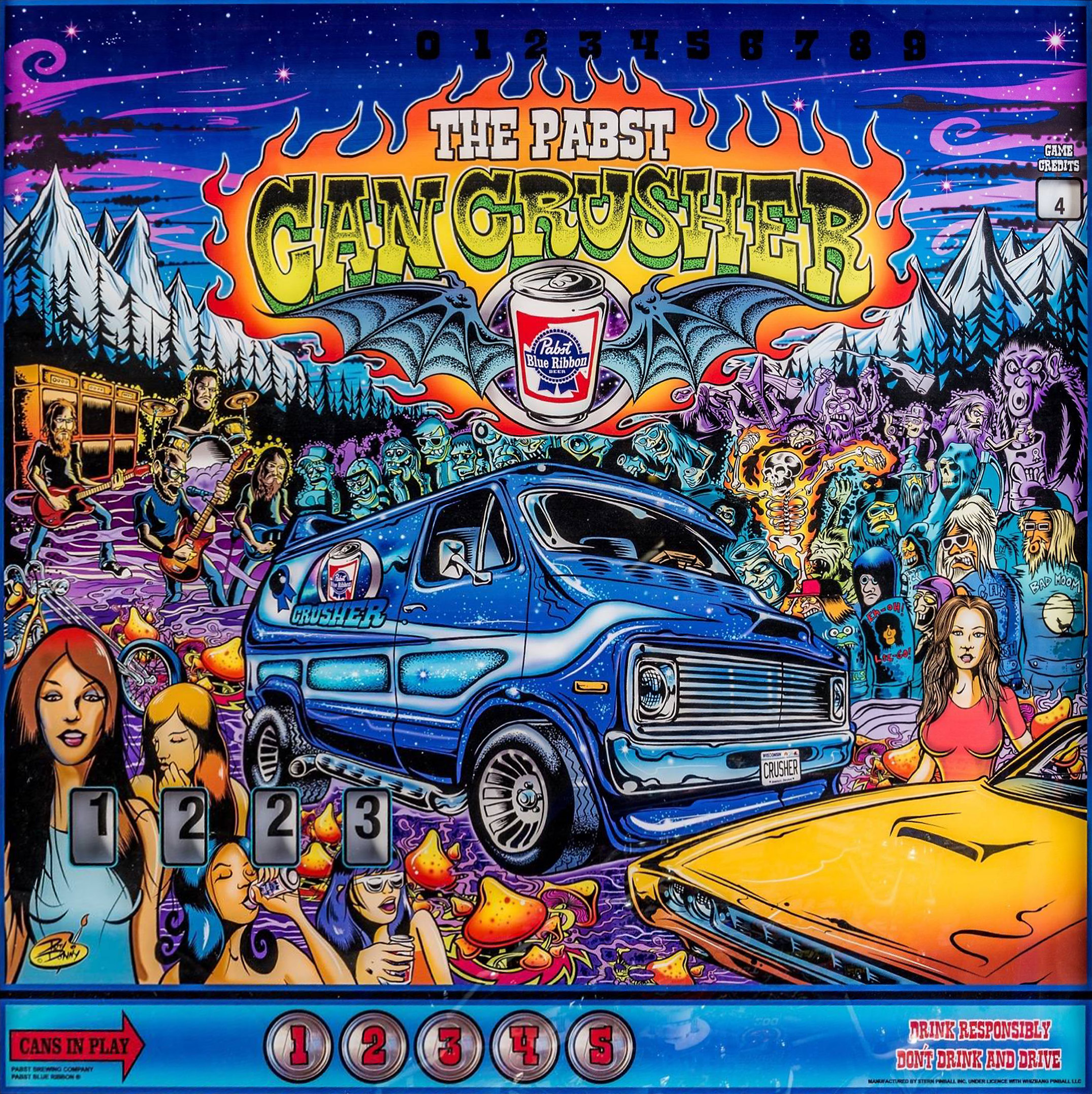This vivid and psychedelic poster from Pabst Blue Ribbon combines vibrant colors with a trippy 70s retro theme. Dominating the center is a blue, galaxy-themed van marked with "Crusher" on both its side and front license plate. Above, an orange and yellow ombre flame frames the headline "The Pabst Can Crusher," with a can of Pabst Blue Ribbon featuring bat wings. The upper backdrop boasts deep blue and purple twinkling skies, snow-capped mountains, and shadowed pine trees, suggesting a nighttime festival or concert scene. Scattered around are eclectic characters: some dancing skeletons engulfed in flames, musicians playing guitars and drums, and colorful-haired women standing behind a yellow muscle car and drinking beer cans. To the right, animals like monkeys or gorillas add a whimsical touch, while mushrooms sprout from the purple ground. The bottom of the poster features the text, "Cans in play, 1, 2, 3, 4, 5, drink responsibly, don't drink and drive," encapsulating the energetic and chaotic nature of the scene.